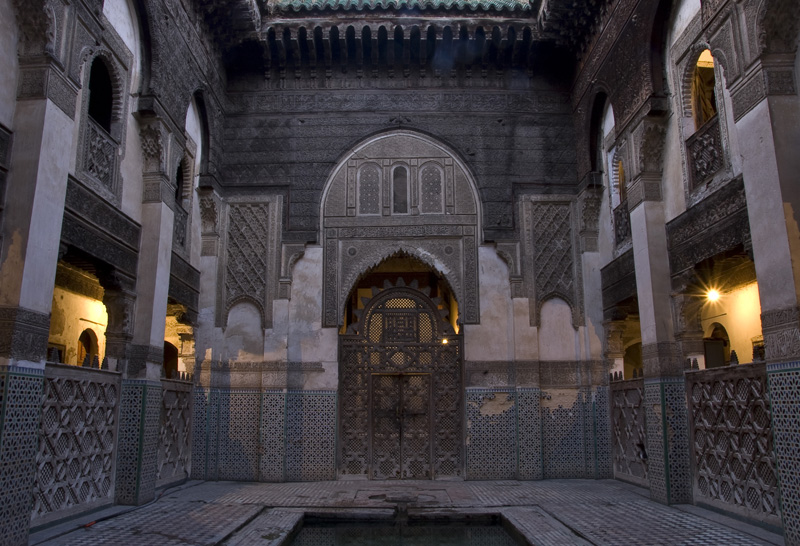The photograph captures the evocative interior of an abandoned mosque, showcasing a rich tapestry of Arabesque architectural elements. Dominating the foreground is a ceremonial ablution pool, once used for ritual cleansing of hands and feet before prayer. The pool's presence, though devoid of water, hints at its past significance. Surrounding the pool are intricately designed geometric tiles that exude the craftsmanship of a bygone era. Adjacent to the pool, a grand iron door stands as a sentinel to the past, its once majestic presence now rusted and weary. Above, a vaulted ceiling stretches out, its arches and patterns drawing the eye upward, symbolizing a connection to the divine. Through the dimly lit interior, partially illuminated exterior hallways can be seen, casting subtle light into the room and highlighting the detailed Arabesque motifs that adorn the walls. The air of neglect is palpable; the space whispers of reverent prayers once offered but now echoes with silence. The overall atmosphere is one of sacred desolation, a once-vibrant place of worship now slowly succumbing to the ravages of time.